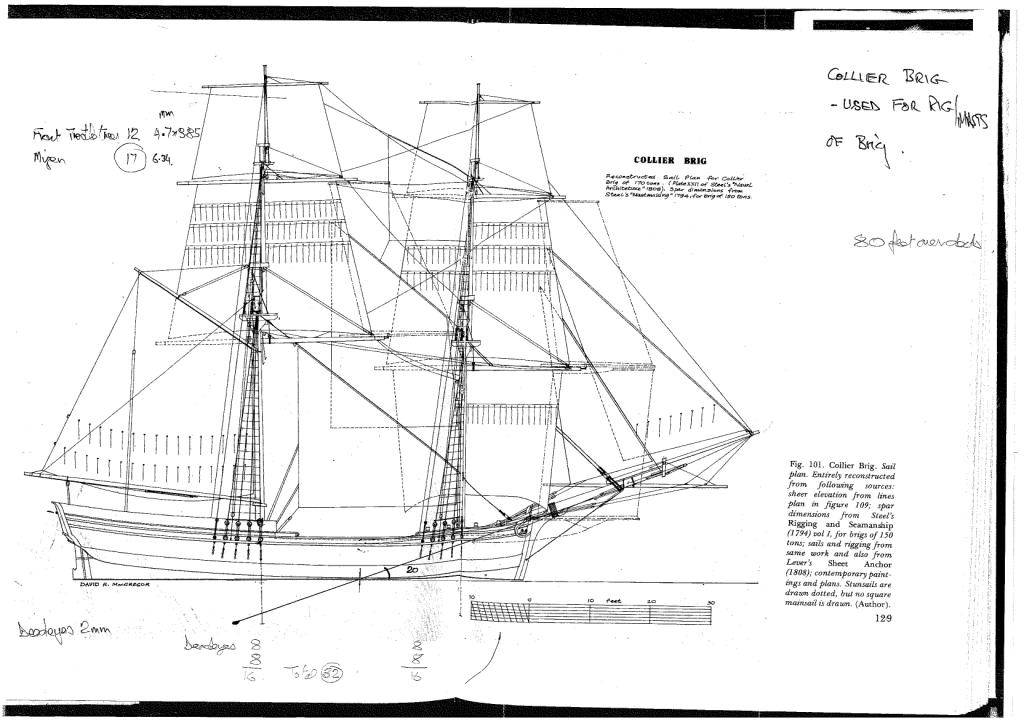The image shows a detailed engineering or design drawing of a pirate ship on a white piece of paper. The ship is oriented to the right in a side view, allowing a clear view of its structure and several sails. The ship features a mast at the front that extends upwards and to the right, and two main poles (masts) positioned centrally on the ship. Each mast features multiple sails of varying sizes, with six or seven sails visible in total. Mathematical equations and notations fill the top corners, with the top right corner containing the text "Collier Brigg used for A.G." Additionally, near the top middle on the right, the phrase "cool cool cool cool life break" is inscribed. Underneath the ship, there are musical staff lines drawn, and in the bottom right corner, there is a small, nearly illegible paragraph ending with "one two nine." More mathematical figures populate the bottom left corner. The entire drawing showcases significant hand-drawn and printed details, highlighting conceptual design elements without specified dimensions.